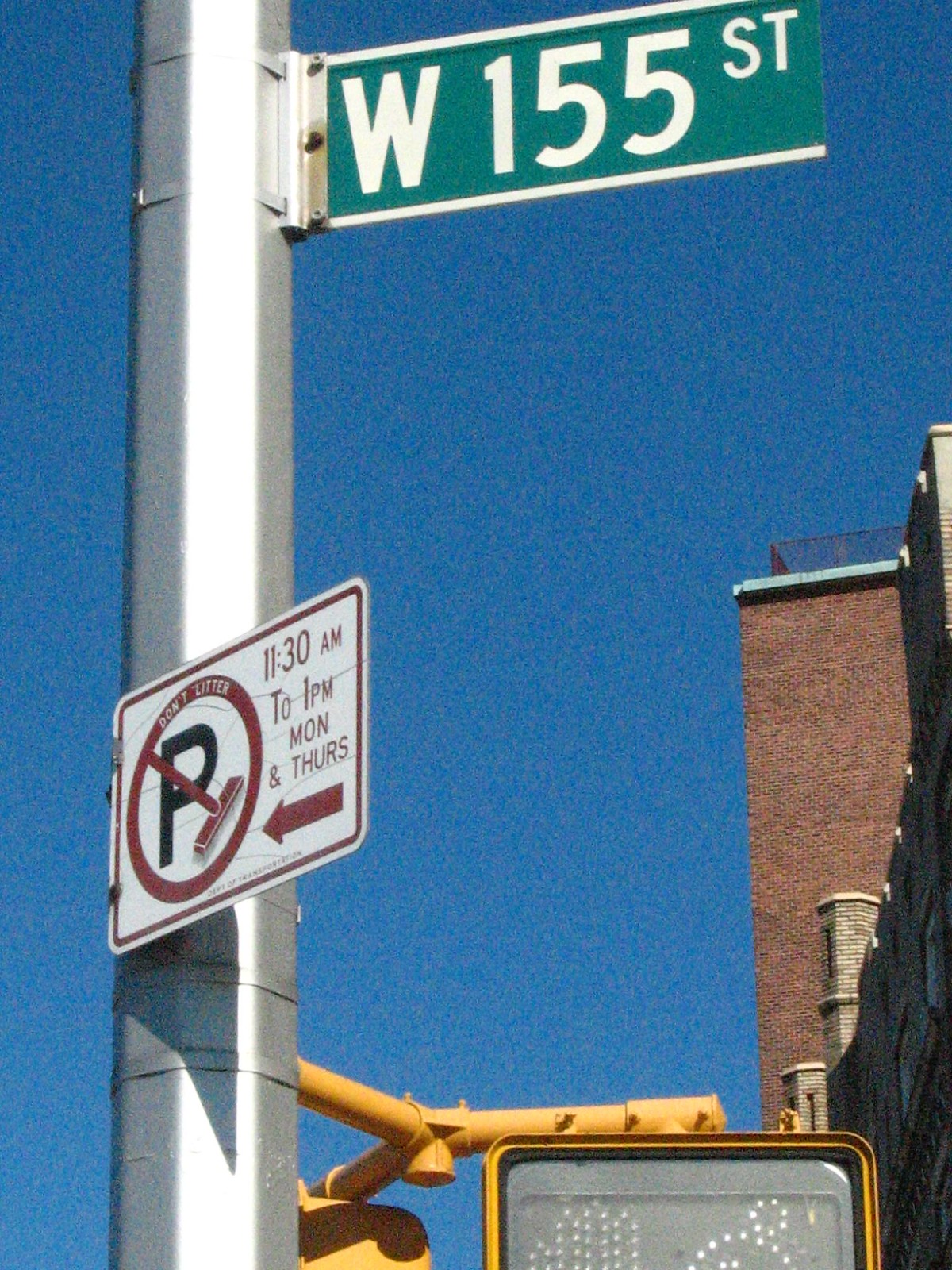The image features a tall metal pole adorned with multiple street signs. At the top, a green sign indicates "W 155 St" in white letters, signifying West 155th Street. Below this, a white sign with bold red and black print details parking restrictions: "No Parking 11:30 AM to 1 PM Monday and Thursday," accompanied by a black "P" symbol crossed out in red and a left-pointing arrow. Beneath this, another sign displays a "No Littering" symbol in red and white. Attached to the base of the pole is a pedestrian crosswalk signal housed in a yellow box on a yellow pole, designed to indicate when to walk or stop, though it appears unlit in the image. In the background, to the right of the pole, a red brick building can be seen, providing an urban context to the scene.